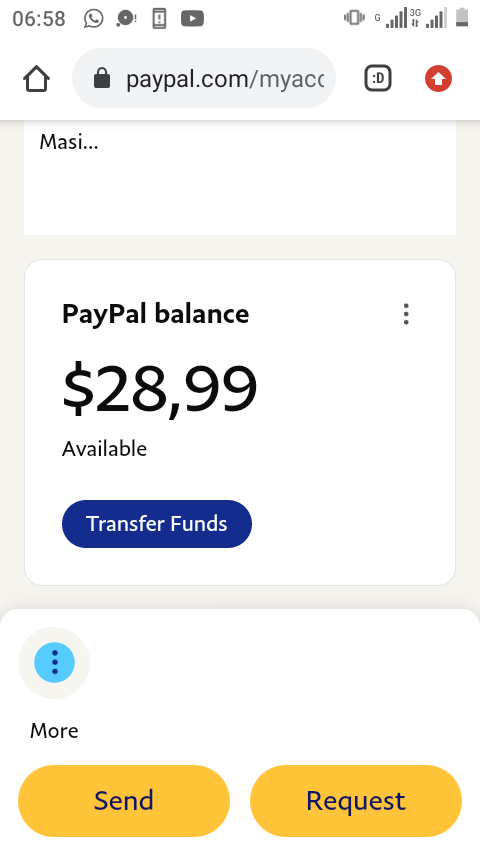This image is a phone screenshot of the PayPal balance screen, displaying various interface elements and details. Starting from the top right, we observe several icons indicative of phone status: a battery icon showing approximately 10% charge, two Wi-Fi signal strength icons – one with 4 out of 5 bars and another with full bars – alongside a phone vibration icon. On the top left, the time captured in the screenshot is 6:58.

Progressing to the top middle, there's a URL bar indicating the website as PayPal.com, flanked by a small square displaying a smiley face emoticon ( :D ) and an upward arrow to the right. Below this area, the central portion of the image shows a prominent box labeled "PayPal balance." Within this box, the available balance is listed as $28.99, and just beneath this, there's a button labeled "Transfer funds."

At the bottom of the image, there are two orange buttons: one on the left says "Send," and the one on the right says "Request." These buttons are designed to facilitate money transfer actions within PayPal.